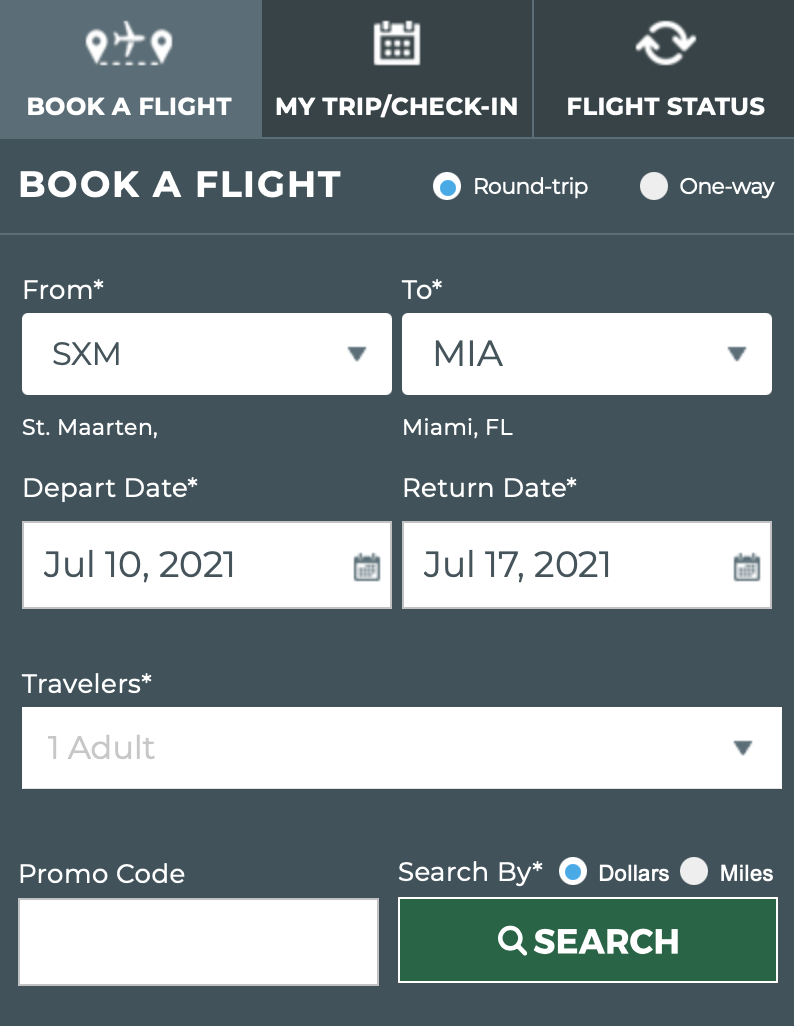This image is a screenshot of a flight booking form from a website with a sleek, dark blue background. The top header is divided into three sections, each labeled with white text and a corresponding logo: "Book a Flight," "My Trip," and "Check-In and Flight Status." Below this header, a second horizontal section features the title "Book a Flight" on the top left. To the middle-right, there are selectable options for "Round Trip" and "One Way," each accompanied by a selection circle.

Further down, the form itself is displayed. The first fields allow users to input the departure and destination locations. Immediately below these fields are sections for selecting the departure and return dates. Continuing down, the form offers options for specifying the number of travelers, denoted as "Travelers" with a drop-down menu or selection tool.

At the bottom left of the form, there is a white box for entering a promo code. On the bottom right, a green rectangle with a white border contains a white magnifying glass icon and the word "Search." Above this search button, there is an option to choose between "Search by Dollars" or "Search by Miles," each with their own selection buttons.